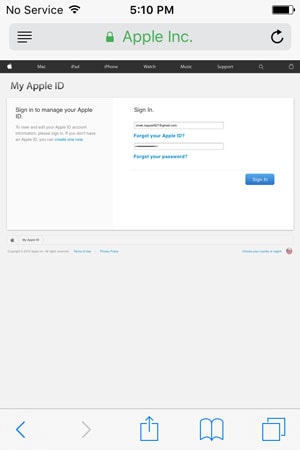The image depicts a smartphone screen displaying an Apple ID sign-in page. At the top left corner, the screen shows "No Service" alongside the signal strength icon. The current time is displayed as 5:10 PM. Below the time, set in a gray box, it reads "Apple Inc." with a green lock icon next to it.

Continuing down, there is a black box displaying the text "My Apple ID" over a grey background. Below this, there is a section prompting the user to "Sign in to manage your Apple ID" with a white box containing further instructions. Within this box, users are instructed to enter their credentials. There are two options in blue text: "Forgot your Apple ID?" and "Forgot your password?" offering help for those who need it. Finally, a blue "Sign In" button is presented for users to proceed.

At the very bottom, amidst a gray background, there are several navigation options: a button on the far left labelled "My Device," a left-pointing blue arrow, a right-pointing gray arrow, an upward-facing blue arrow on a page icon, a blue split-screen icon, and a blue icon representing two overlaying pages.

The detailed layout and color scheme provide a clear and structured interface for managing an Apple ID account.